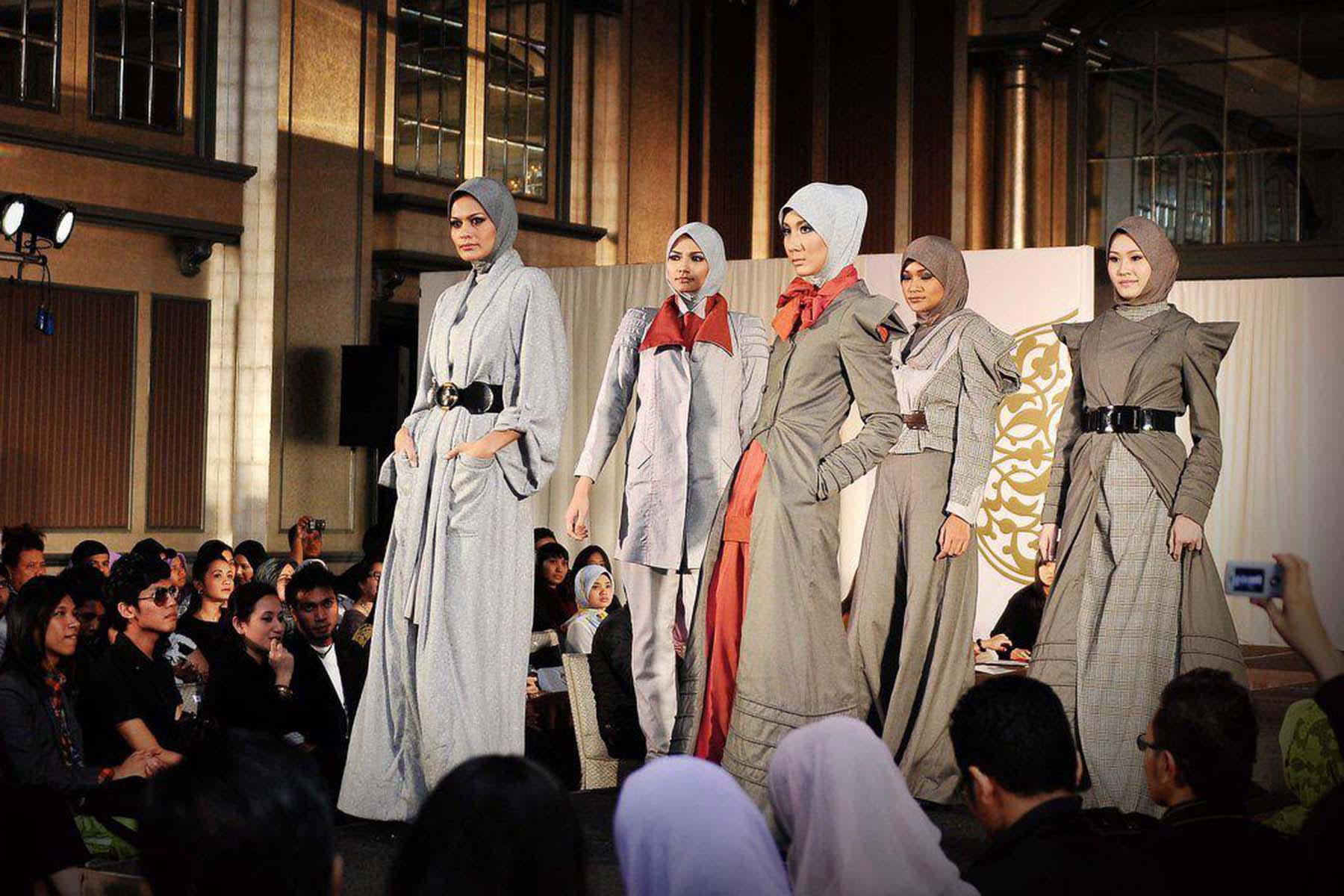This photograph captures a solemn moment at a fashion show, featuring five Muslim women confidently modeling on a raised runway. The women are dressed in long, neutral-colored coats and dresses predominantly in shades of gray and beige, accented by black belts. Notably, one woman stands out in a reddish-orange outfit under a gray jacket. All the women are wearing hijabs, adding to the cohesive, modest aesthetic. Their serious facial expressions convey a sense of strength and resilience. In the background, the setting appears industrial, with tall brown walls, high windows, and possibly mirrored surfaces, enhancing the scene's grandeur. On both sides of the runway, an attentive audience of men and women captures the moment with cameras, adding to the event's professional atmosphere.